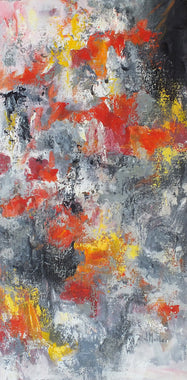This image showcases a small, rectangular canvas painting, held in an upright portrait mode. It is an abstract artwork dominated by a chaotic blend of colors including distinct splashes of red, orange, yellow, and hints of pink, all merging over a base of white, black, and gray. The painting features random brush strokes and smudge patterns, creating an unstructured, dynamic feel without any discernible subject. The top of the canvas has a darker spot, with the hues lightening towards the bottom and the left, enhancing the complexity and fluidity of the artwork. The vibrant splatters of red, orange, and yellow give an impression as if flower petals were thrown onto a wet surface, further contributing to its intricate and imaginative nature.